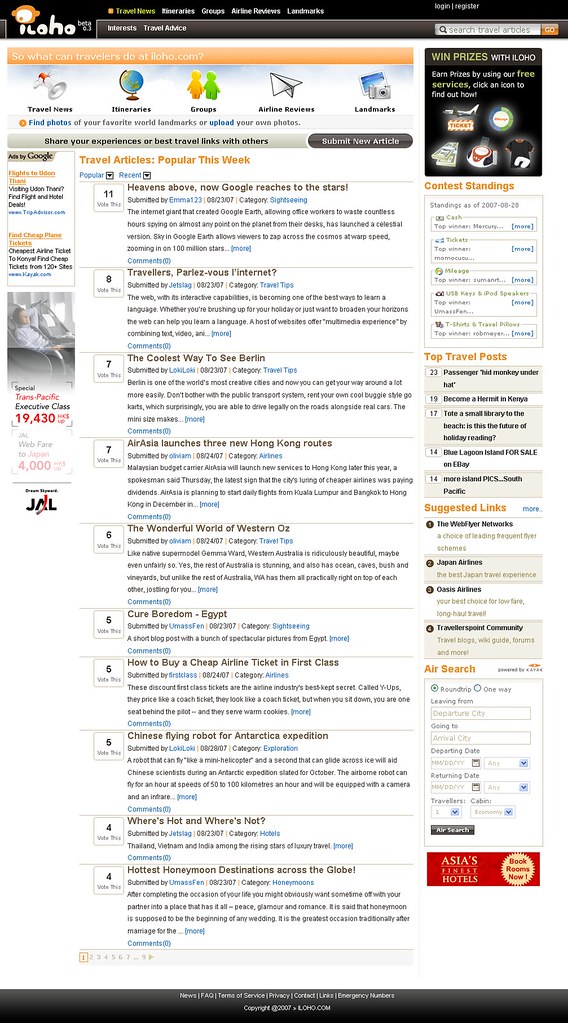This image is a screenshot of a website titled "ILOHO," identifiable by the logo positioned in the upper left-hand corner, which features a stylized monkey head with a dot for an eye. The website seems to focus on travel, showcasing a section titled "Popular Travel Articles This Week" prominently at the center. This section lists ten articles:

1. "Google Reaches to the Stars"
2. "Traveler's Pal: A View on Internet"
3. "The Coolest Way to See Berlin"
4. "Air Asia Launches Three New Hong Kong Routes"
5. "The Wonderful World of Western Oz"
6. "Cure Boredom"
7. "How to Buy a Cheap Airline Ticket in First Class"

Each article headline suggests a diverse range of topics related to travel, from tech innovations to destination guides, airline news, and tips for savvy travel.